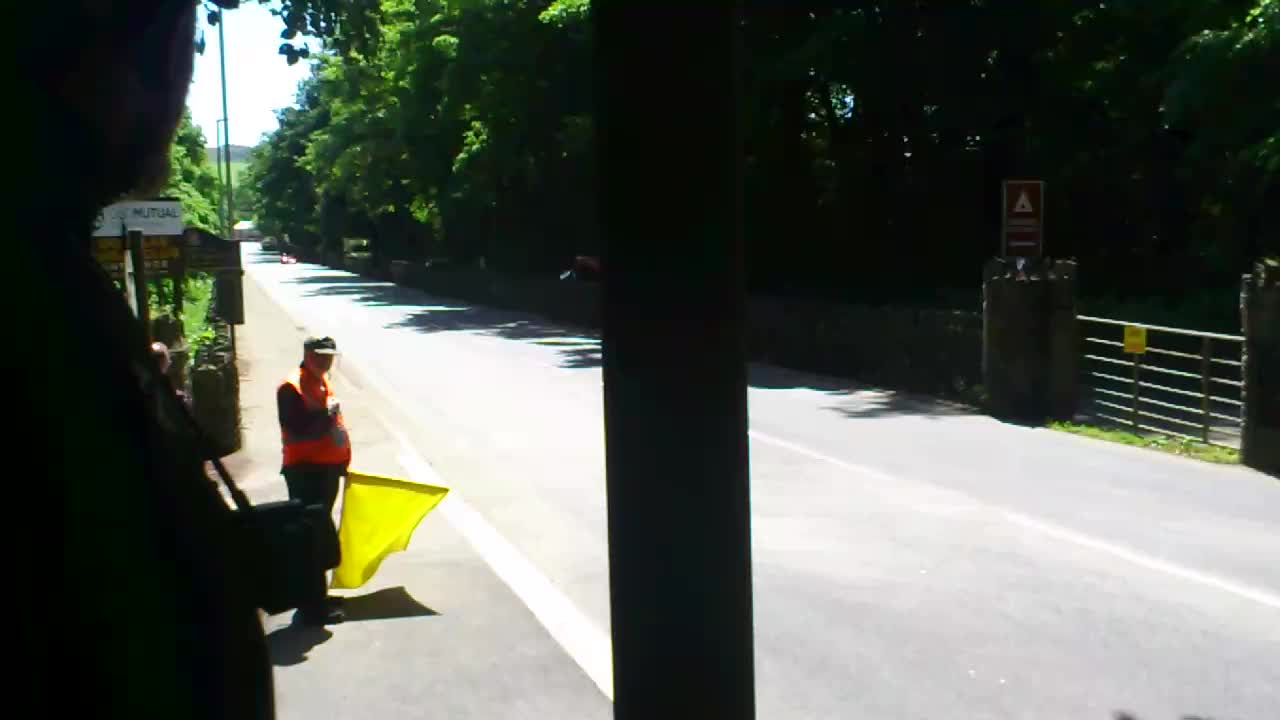The photograph depicts a quiet country road bathed in sunlight, bisected by a tall telephone pole at the center. The crossing guard, dressed in a bright orange vest and a baseball cap, stands on the shadowed side of the street, holding a large, vivid yellow flag. He gazes down the near-empty road, which stretches into the distance flanked by lush green trees with overhanging branches casting shadows on the pavement. Across from him is an iron gate connected to cement columns. A distant figure on a bicycle and additional telephone poles lining the left side of the road contribute to the tranquil, almost surreal atmosphere of the scene.